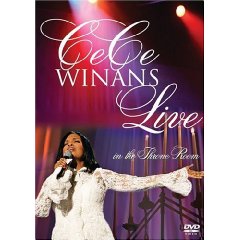The DVD cover prominently features a live performance by C.C. Winans. The top half of the cover displays the title "C.C. Winans Live" in bold white lettering against a backdrop of a red curtain illuminated by several spotlights. In the bottom half, a striking photograph captures C.C. Winans mid-performance. She stands with her left arm outstretched and her right arm bent at the elbow, holding a microphone close to her face. Winans is dressed in an elegant, long-sleeve, lacy white blouse that buttons up at the front, with wide, loose sleeves that add a dramatic flair to her extended arm. Her long, black hair cascades behind her as she sings passionately. Adding a touch of theatrical ambiance, a purple curtain serves as the background, along with an edited-in image of a candelabra behind her extended arm. The bottom right corner of the cover appears to have some small, partially obscured text, which includes "D.B.D."